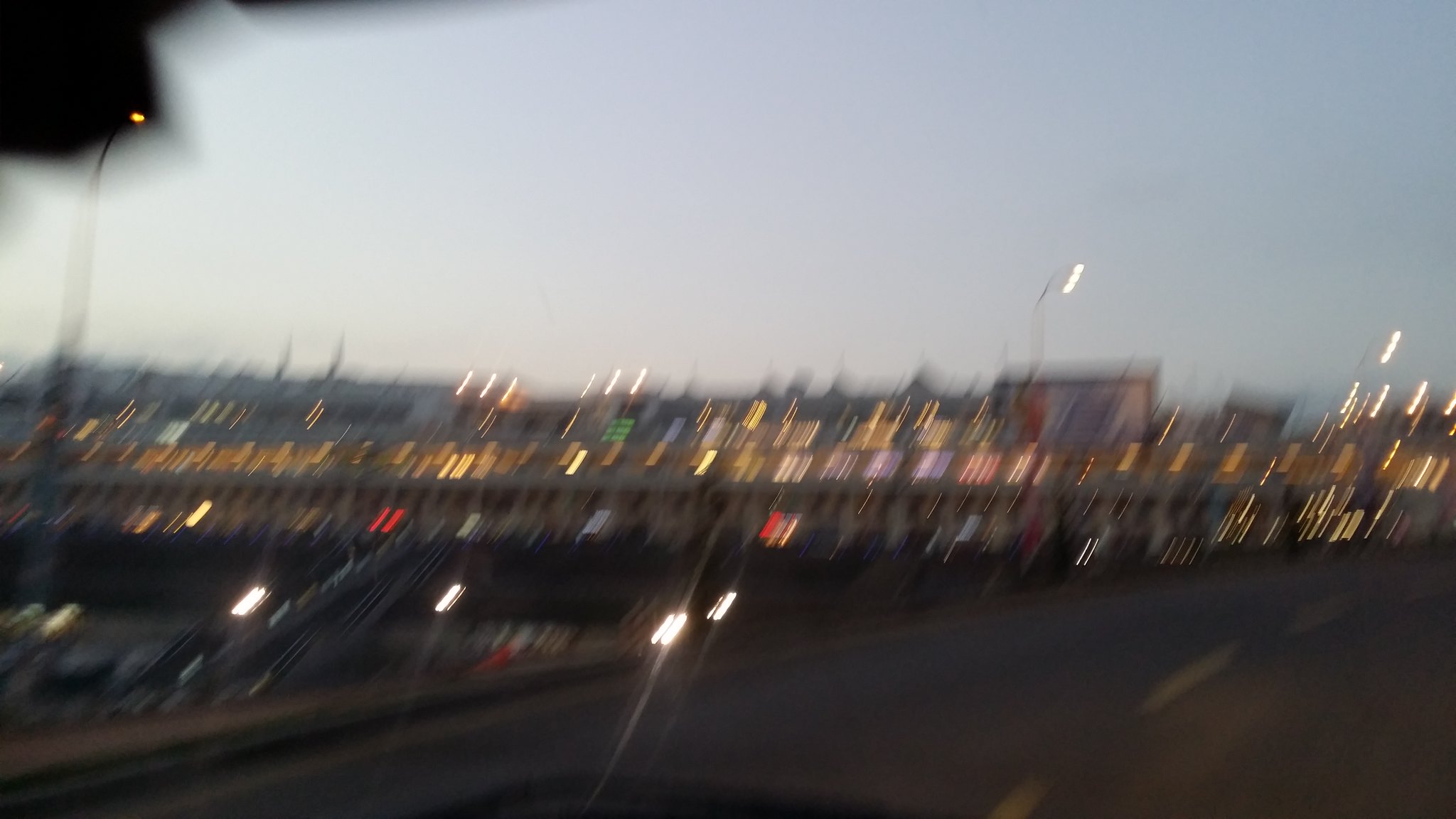A blurry landscape photograph taken from a moving car on a highway at dusk. The rectangular image captures a portion of the black car in the upper left corner. The dark gray road features yellowish-white lines. In the background, various businesses are visible, adorned with lights in shades of yellow, white, red, green, purple, and pink, all set against a grayish sky. The blurred effect adds a sense of motion and evening ambiance to the scene.